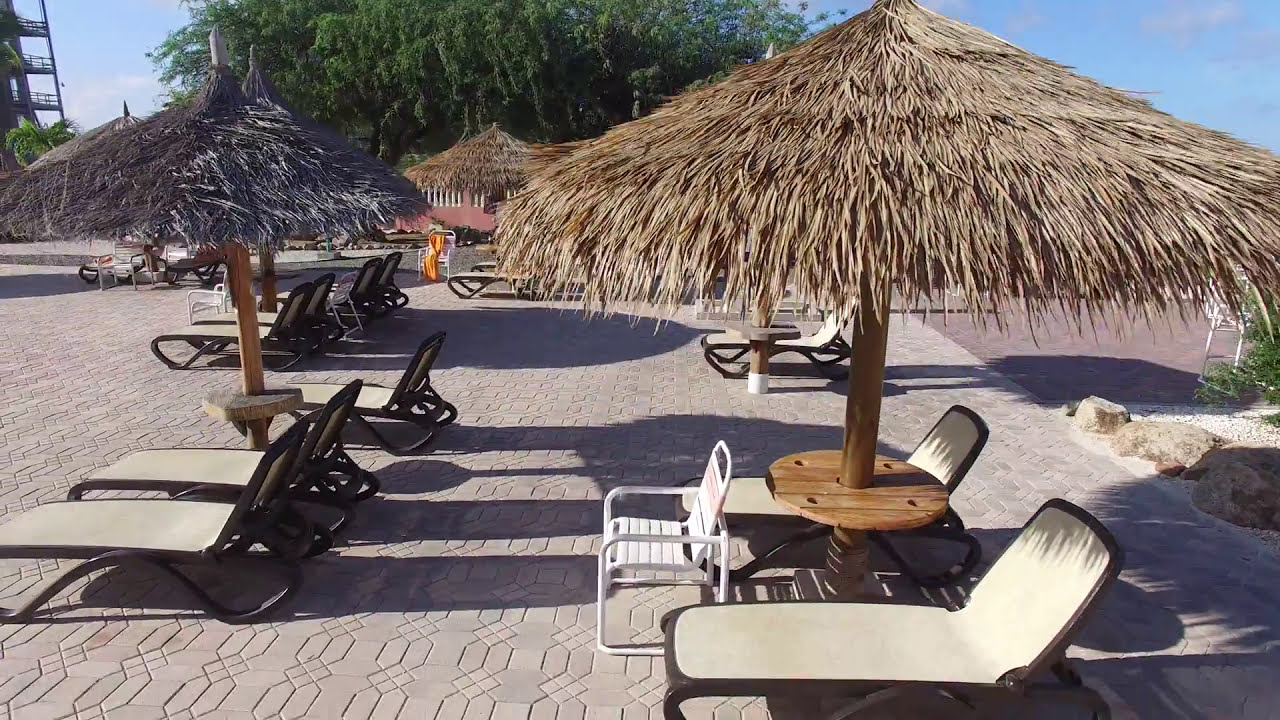The image depicts a serene, inviting scene at an exotic resort, characterized by a neatly organized assortment of tan and brown-framed beach chairs and chaise lounges arranged on an expansive patterned gray stonework ground. At the center-right, two tan beach chairs flank a brown thatched umbrella with a wooden post, complemented by a small wooden table in between. In front of these chairs, a single white, non-reclining beach chair is placed. This setup is mirrored in several other groupings of chairs and thatched umbrellas extending towards the left side and into the distance. The bright blue sky with scattered clouds adds a tranquil backdrop, further enhanced by a large green tree with lush leaves in the distance. On the right side of the background, the stone tiles shift to darker hues, suggesting a walkway bordered by rocks and red brick. The left upper corner features what appears to be a tower with multiple staircases or scaffolding, contributing a touch of architectural intrigue to the resort's landscape.